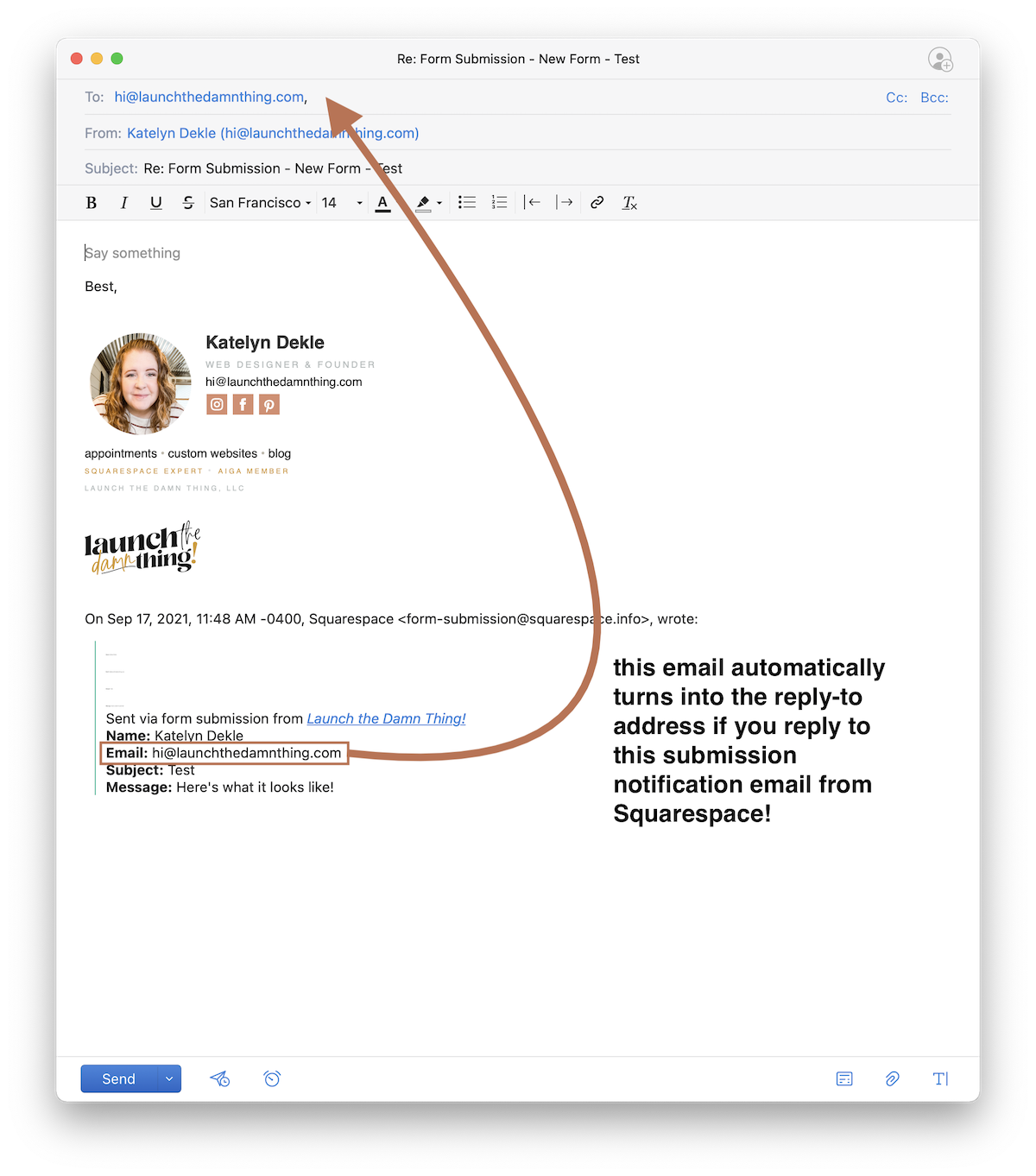**Email Screenshot Description:**

The screenshot captures an email interface. At the top, there's a light gray header divided into cells, and above this header are three small, circular buttons in red, yellow, and green, typically used for window control in certain operating systems. The email is titled "Ray Form Submission, New Form - Test," displayed centrally at the top.

On the right side of the header, there's a circular profile icon. Below this is the main body of the email with the following details:

- **Recipient**: The recipient's name is in blue font next to the label "To."
- **Sender**: Caitlyn Diecky is identified as the sender, with her name and email address displayed in blue font.

The subject line reads "Ray Form Submission, New Test - Test" in black font. Directly below the subject line, there's a toolbar with widgets for formatting options such as bold, italic, underline, font changes, and color changes.

The message starts with the text "Buy something" followed by "Best," and then the sender's signature. The signature includes a profile photo of a fair-skinned woman with curly red hair wearing a striped shirt. Her name, Caitlyn Diecky, is in bold next to the photo, along with her email address and social media icons.

Following this, another piece of text reads, "Launch the dang thing."

The email thread underneath shows a previous email dated September 17, 2021, at 11:48 AM (0400) from Squarespace's form submission service. The previous message notes that it was sent via form submission with the subject "Launch the damn thing" and lists Caitlyn Diecky as the sender with her email address. The text has a red box around it with a long arrow pointing toward the "To" line above, indicating the relation between the messages.

On the right-hand side, in lowercase bold font, there’s a note stating, "this email automatically turns into the reply-to address if you reply to this submission notification email from Squarespace."